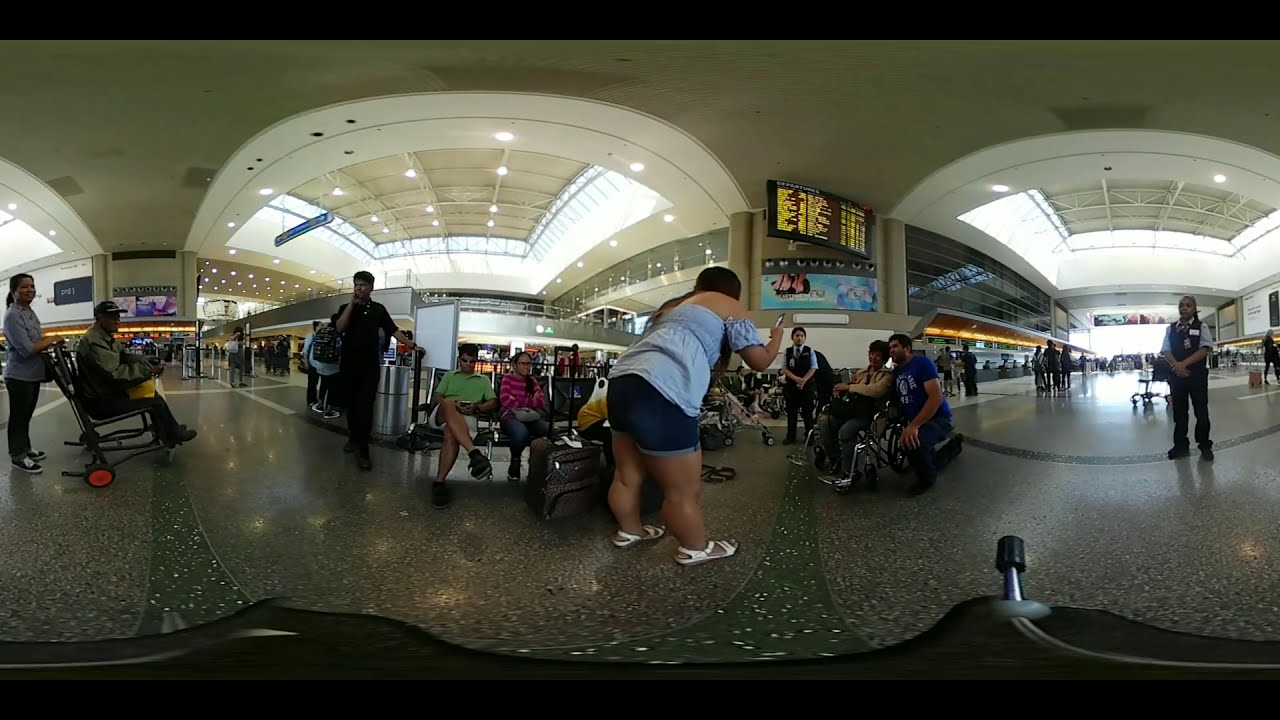The image depicts a bustling indoor scene, likely set in an airport or transportation hub, captured with a fisheye lens. The floor is a shiny, dark tile surface, reflecting the overhead lights and natural sunlight streaming through ceiling windows. In the center of the image, a young woman wearing dark blue short pants and a light blue off-the-shoulder top with white sandals is bent over, possibly examining her luggage. Behind her, various pieces of luggage are visible. Nearby, another woman in blue jeans and a similar light blue top is taking a picture of a person in a wheelchair, accompanied by someone kneeling beside them. To the left, a man sits in a rocking chair with a female standing behind him. The scene is lively with several people walking around and sitting, hinting at the busy, transient nature of the location. In the distance, lines and counters can be seen, flanked by a couple of businesses, adding to the atmosphere of an active, daytime indoor setting. The palette of the image includes black, gray, white, tan, shades of blue, green, pink, red, and orange, contributing to the vibrant yet functional design of the space.